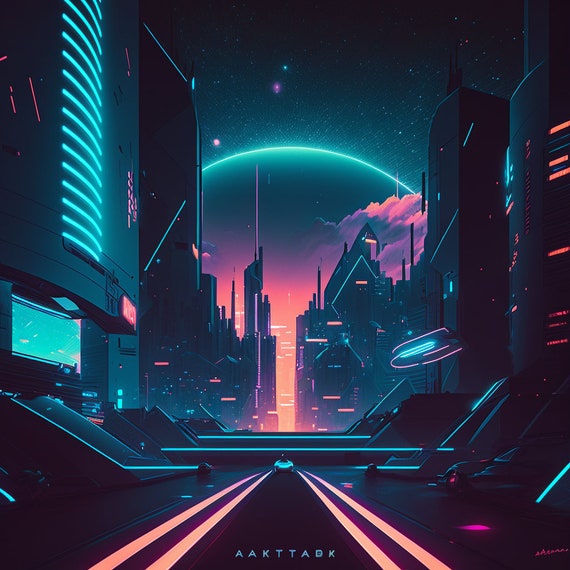The image is a vibrant piece of digital art showcasing a futuristic, cyberpunk cityscape bathed in neon colors. Bright cyan, orange, pink, and blue hues contrast sharply against the dark background, creating a striking visual effect. In the foreground, two bright pink lines resembling road markings lead into the distance, flanking a small, neon-green vehicle. Below these lines, the text "AAKTTABK" is written in small blue letters. To the right of this text, there is a pink signature. The city skyline features buildings illuminated with neon cyan and orange lights, and above it, a gradient-filled sunset fades into a sky adorned with scattered stars. A celestial arc, possibly representing a planet or moon, with a neon light blue ring, looms large over the city, enhancing the otherworldly atmosphere.